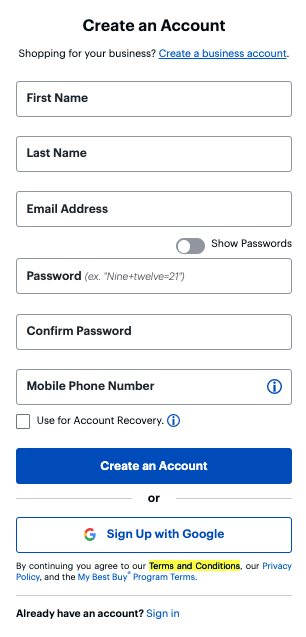This image is a cropped screenshot of the "Create Account" screen on Google. The rectangular panel is centrally focused, and the top displays "Create an Account" in bold black font. Below this, "Shopping for your business" is listed in smaller black font, with a blue hyperlink reading "Create a business account" to the right. 

The form consists of several vertical text boxes for user input: the first one is labeled "First Name," followed by "Last Name," and "Email Address." Adjacent to the email address field on the right, a toggle button marked "Show Passwords" is switched off. Below, there are three additional fields for "Password," "Confirm Password," and "Mobile Phone Number." Next to the mobile phone number field is a checkbox labeled "Use for account recovery."

At the bottom, a large blue button features the text "Create an Account" in prominent white letters. Directly beneath this, centered, is the word "or." A secondary large button displays the Google logo on the left with the text "Sign up with Google." At the image's very bottom, a small-sized disclaimer in black font includes the term "Terms and Conditions," highlighted with an edited yellow background.